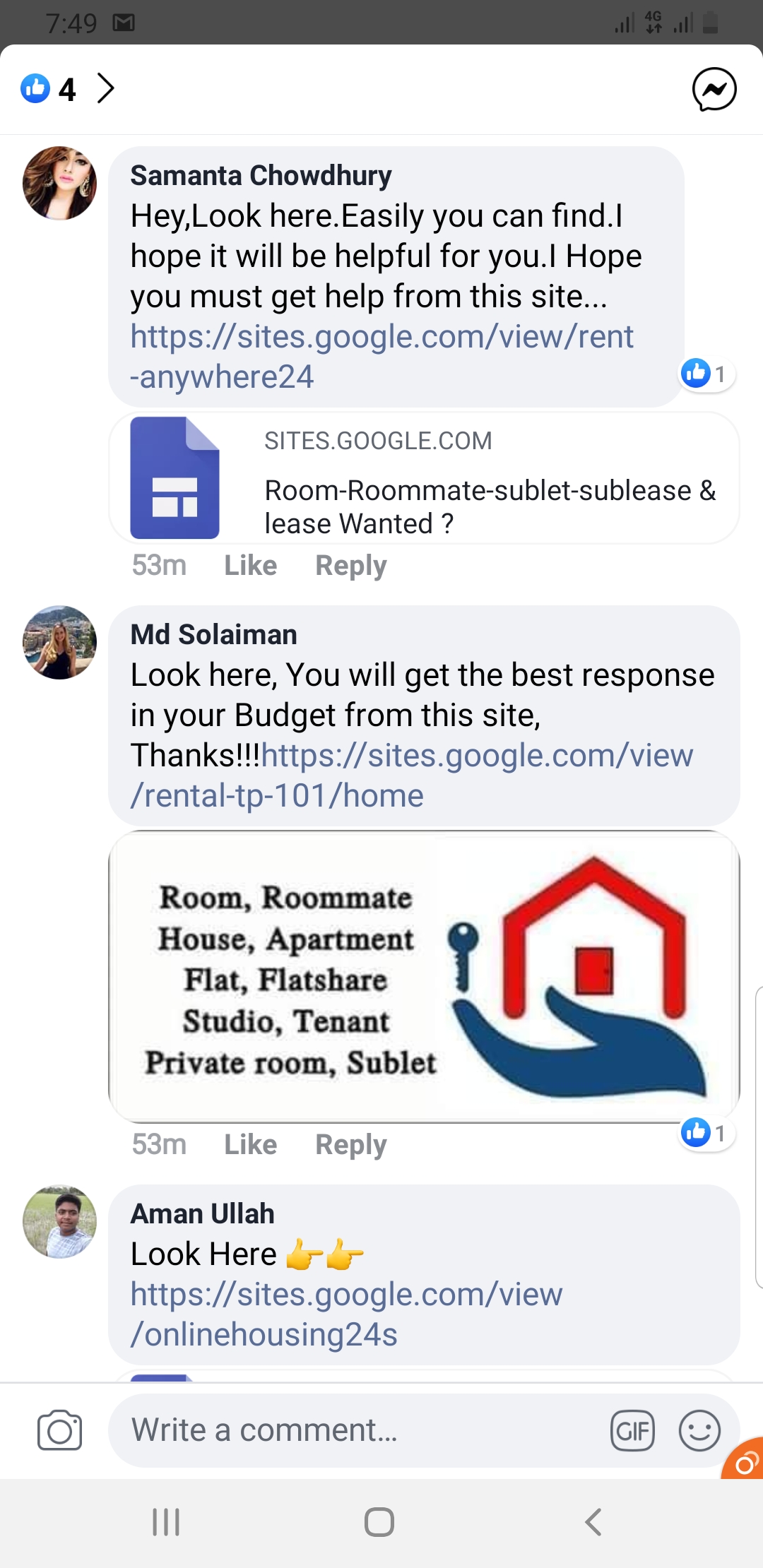This image is a screenshot taken from an Android device. At the top, a faded gray notification banner displays the time as 7:49 AM and includes a Gmail icon. On the right side, there is a nearly full Sigma bar, followed by another faded icon that is difficult to identify, and then another Sigma bar. The battery icon, which is about a quarter full, is also visible here.

Overlaid on the screen is a thumbs-up sign inside a blue circle, next to the number 4 and a right-pointing arrow. To the left, there is a circle with a lightning bolt inside it. Below this, a user profile picture of a lady is displayed along with the name "Samantha Chowdhury" (C-H-O-W-D-H-U-R-Y). Her message reads: "Hey look here, easily you can find. I hope it will be helpful for you. Hope you must get help from this site. Hope you must get it." Following her message is a URL: sites.google.com.

Beneath Samantha's message is another user message with a profile picture. This section includes additional information and a response. A website icon is present, followed by icons and text related to roommates and housing options, specifically mentioning room, roommate, house, apartment, flat, last year, studio tenant, private room, and sublet.

At the bottom, there is another profile icon accompanied by the name "Aman Ullah," along with a message saying "look here" and a subsequent website link.